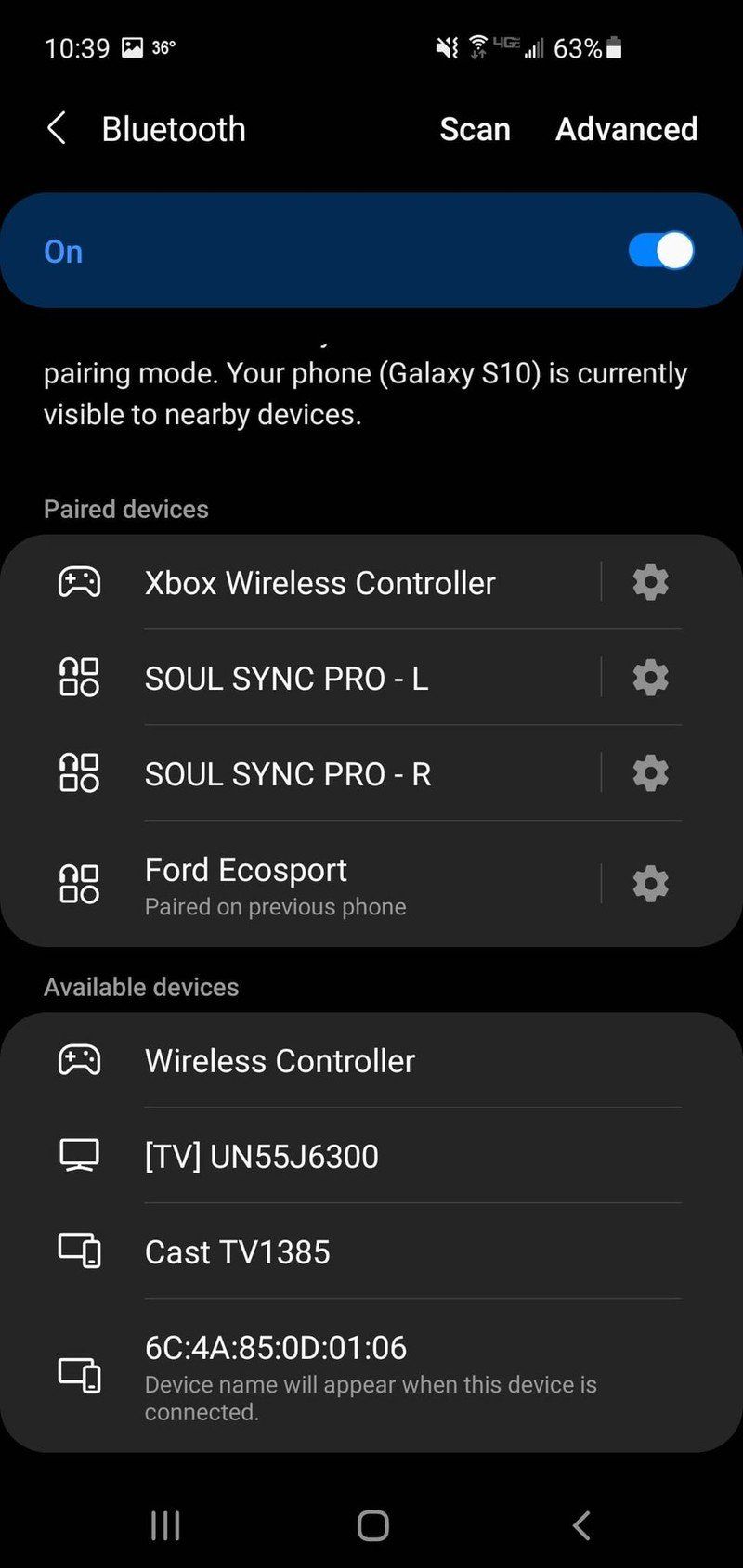Here is a meticulously detailed and cleaned-up caption for the described image:

---

The image depicts a mobile device screen focused on Bluetooth settings. The top portion features a black background, a blue toggle button indicating that Bluetooth is "On," and a note below stating "Pairing mode: Your Galaxy S10 is currently visible to nearby devices." The screen is divided into three sections.

The first section entitled "Paired devices" lists:
1. Xbox Wireless Controller
2. Sol Sync Pro - L
3. Sol Sync Pro - R
4. Ford EcoSport (labeled as paired on a previous phone)

The second section, labeled "Available devices," includes:
1. Wireless Controller (similar to the Xbox controller listed above)
2. TV UN55J6300, indicated by a small TV icon, with the casting option labeled "Cast TV"
3. An unidentified device with a long alphanumeric string

The screen's predominant colors are black and gray, with white text for easy readability.